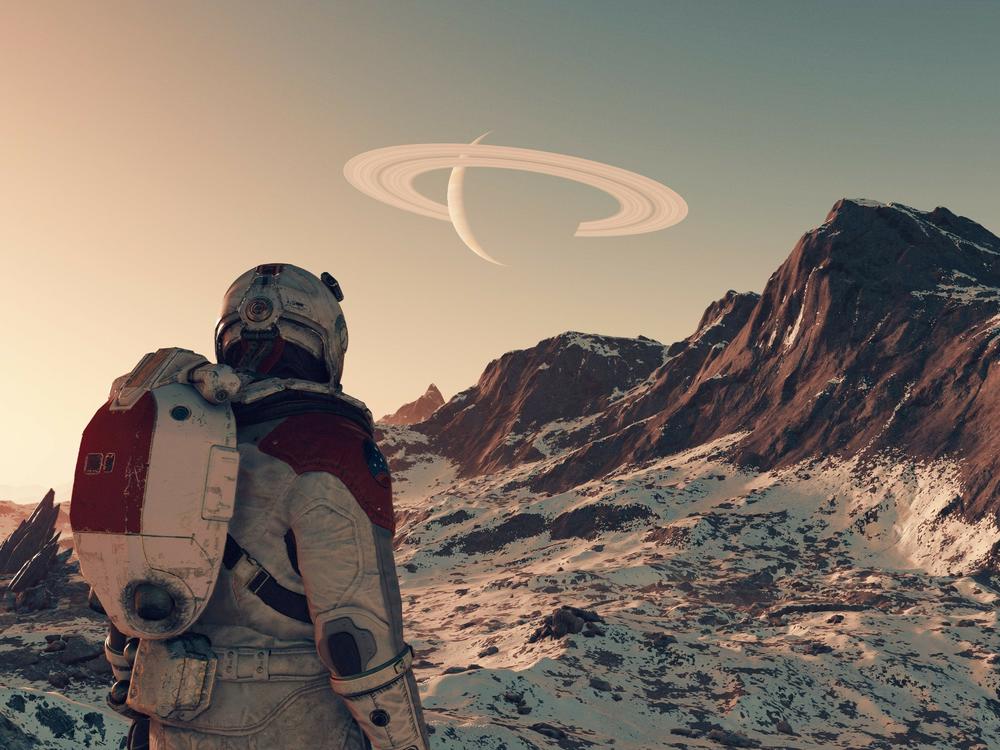In this computer-generated image, an astronaut wearing a distinctive red and tan space suit with a backpack, presumably for oxygen, and dark elbow pads, stands on a snow-covered, barren terrain filled with rocky and bumpy brown mountains. The astronaut is gazing up at a striking view of Saturn with its iconic rings prominently displayed in a sky that offers an intriguing mix of orange, teal, and turquoise hues. The scene conveys a sense of solitude and curiosity, as the astronaut appears to be surveying an alien, yet eerily beautiful, landscape devoid of any text or writings.